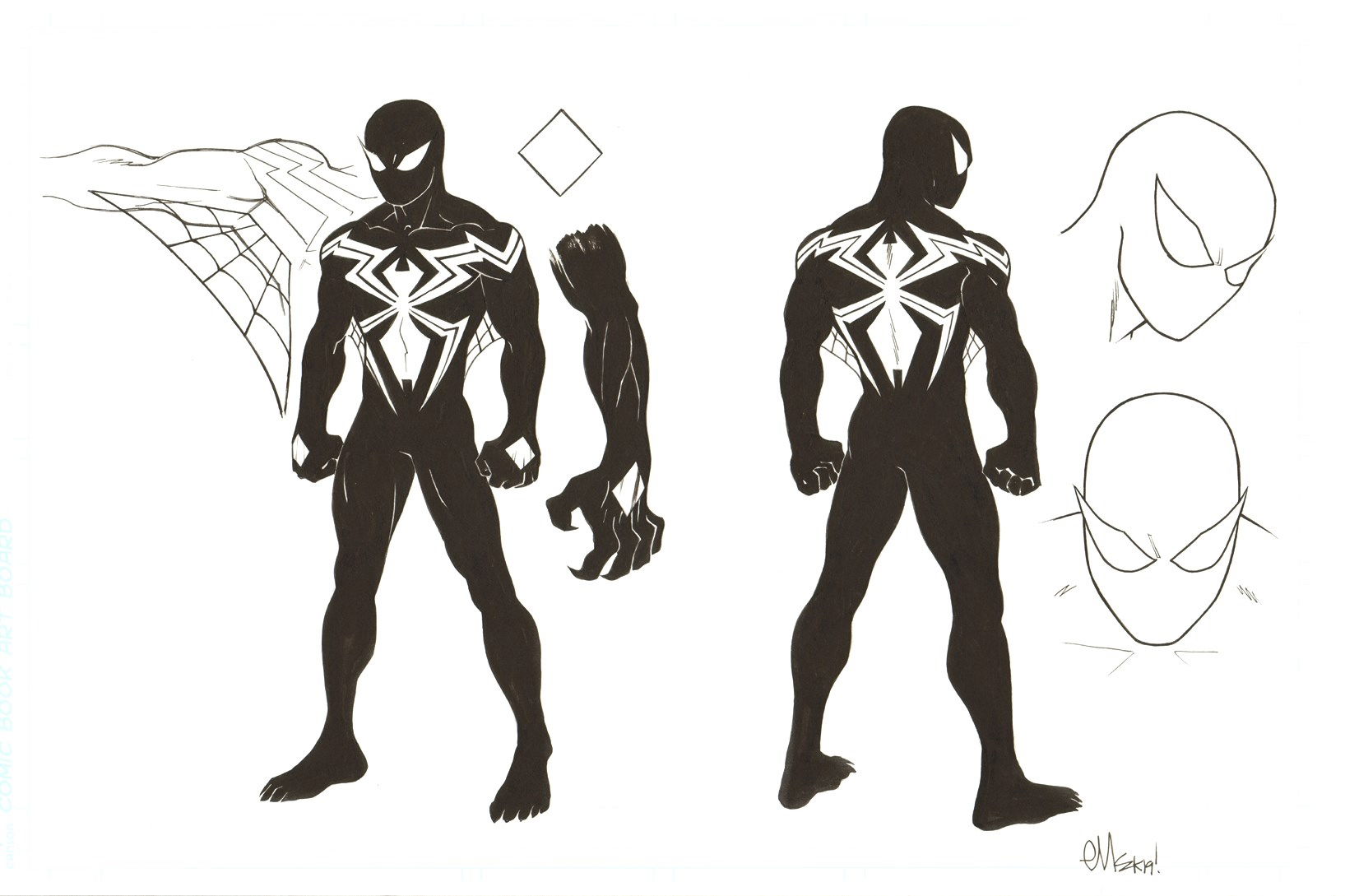The detailed concept art image features a superhero character from the Spider-Man universe, specifically Venom. The illustration showcases Venom from various angles, displaying both his front and back views. The left section of the image presents a frontal view, highlighting Venom's muscle-bound physique clad in a black, skin-tight one-piece suit. Prominently featured on his chest is a large, white spider emblem. His arms display white diamond-shaped patterns on the backs of his gloves, each adorned with long, sharp talons. A close-up reveals an intriguing detail—a web-like material stretching in his armpits. The eyes of Venom are sharply angled, bright white, and extend outward menacingly.

The right section of the image depicts Venom from behind, where he has a matching white spider emblem similar to the one on his chest. Additionally, there are close-up sketches of his head showing his menacing eyes and sharp features. The artwork is rendered entirely in black and white, enhancing the contrast between the dark suit and the bright white details. In the bottom right corner, the artist has signed the piece with the initials "E.M.S.K.A."